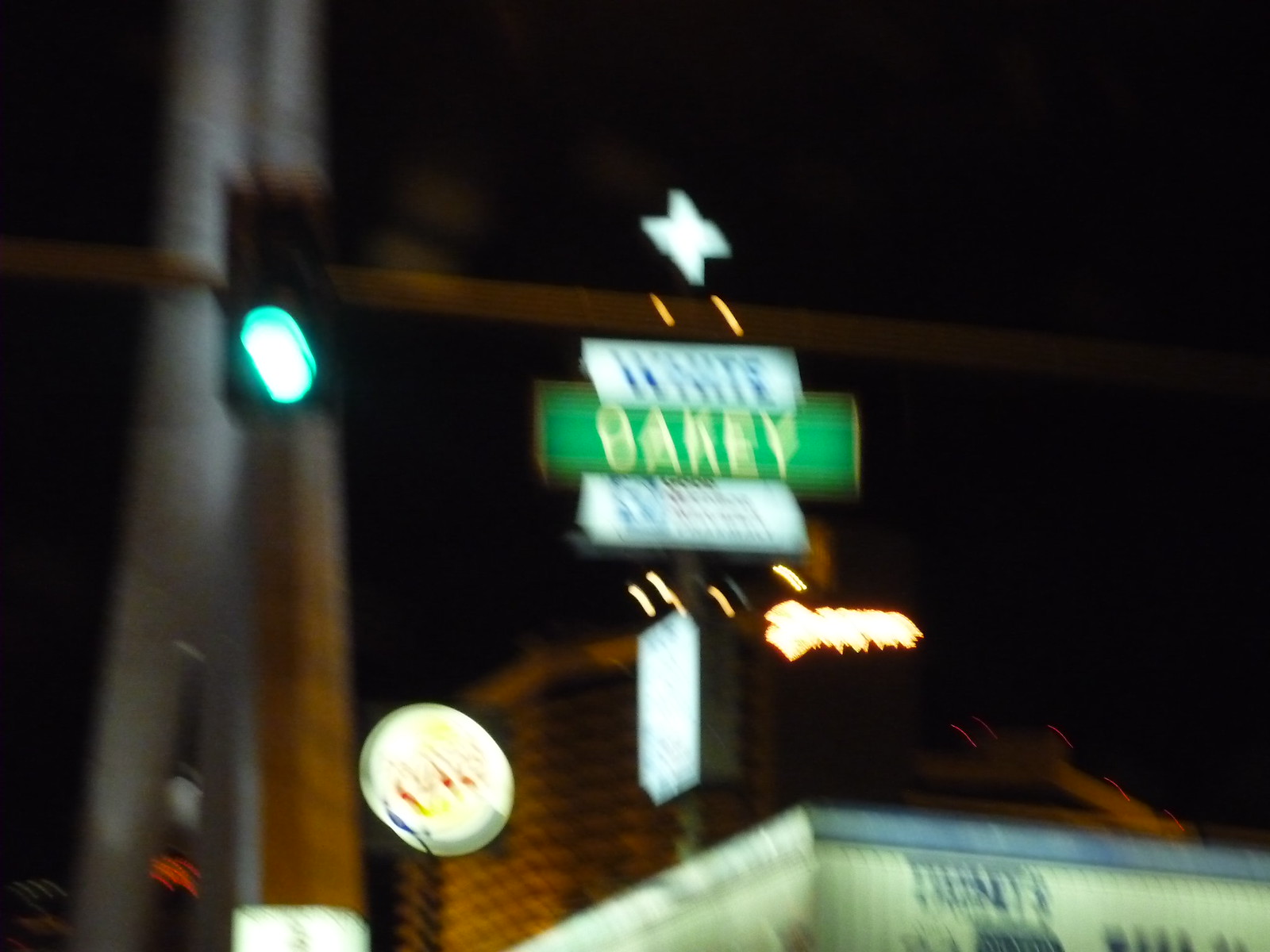The image depicts a highly blurred urban landscape centered around various signs. Dominating the middle is a green sign adorned with white letters, though its text remains unreadable due to the blur. Above and below the green sign are segments of another white sign. To the lower right, a marquee-like sign seems to be advertising a movie or play, with the discernible word "presents." The background reveals a potential high-rise building in muted brownish-beige tones, surrounded by numerous indistinct bright lights. The overall effect is an amalgamation of city elements, merging into an almost abstract scene primarily defined by its unfocused details.